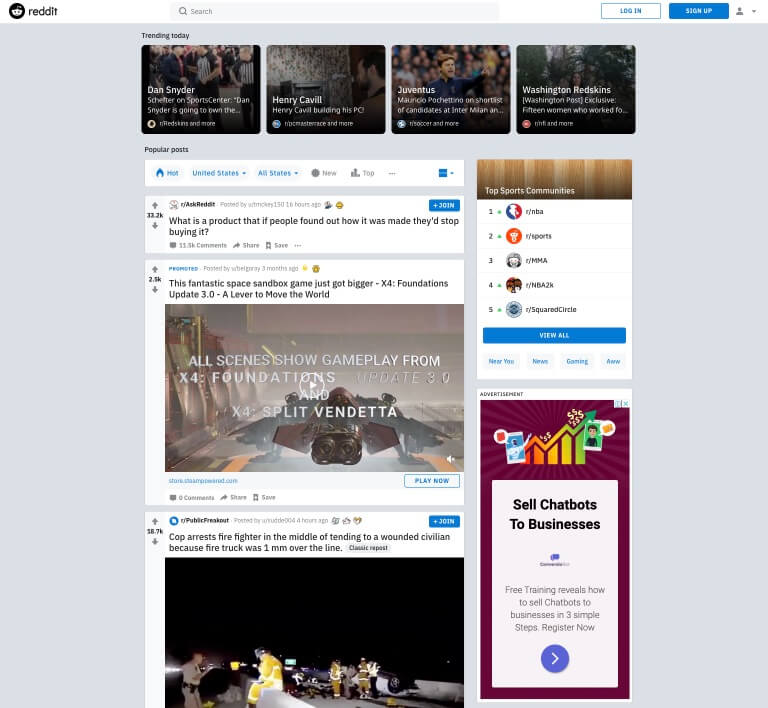**Detailed Caption for Reddit Screenshot:**

A screenshot of a user's main page on Reddit, highlighting various elements and trending topics. At the top, there's a "Trending Today" section featuring topics such as Dan Snyder, Henry Kassel, Juventus, and Washington Redskins. In the upper right-hand corner, there are options to log in or sign up: one button with a blue background and white lettering, and the other with a white background, blue outline, and blue lettering.

The page is divided into sections, starting with "Popular Posts." The first post is from the subreddit r/AskReddit with the question, "What is a product that people stopped buying after finding out how it was made?" Below this is a promoted advertisement for the game "X4 Foundations Update 3.0," highlighting a fantastic space sandbox experience. The scenes shown feature gameplay from the new update.

Further down, there's another post from the subreddit r/PublicFreakout, detailing an incident where a cop arrested a firefighter who was in the middle of aiding a civilian because the firetruck was slightly over the line. The user expresses anger at the cop's actions.

The bottom section lists top sports communities, including subreddits r/NBA, r/Sports, r/MMA, r/NBA2K, and r/SquaredCircle. An advertisement for selling chatbots to businesses is positioned in the bottom right-hand corner of the screen.